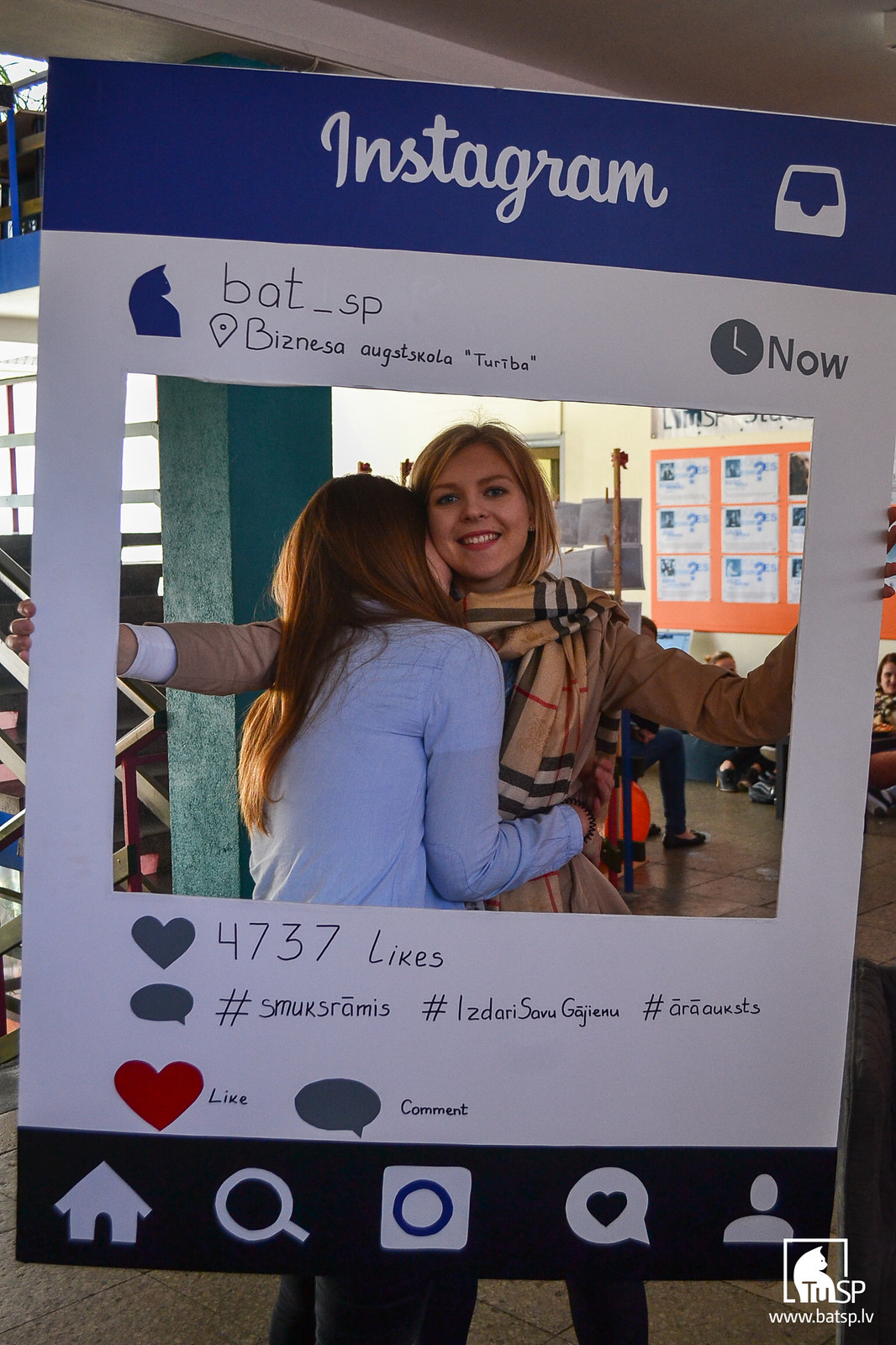This photograph captures two young women, possibly in their early 20s, staging a live replica of an Instagram post. They are holding up a large cardboard frame designed to look like an Instagram interface, complete with the iconic blue banner and white lettering spelling "Instagram." The setup includes various other details such as hashtags and a like count showing 4,737 likes.

The women are dressed warmly, suggesting the weather might be cold. The woman on the left, who has long brown hair, is wearing a light blue shirt and pants. She is partially obscured as she buries her face in a hug with the woman on the right. The woman on the right has blonde hair and blue eyes, and she is dressed in a coat, possibly a raincoat, with a scarf. She smiles slightly as they pose, both framing their faces within the Instagram-like cardboard cutout. 

The detailed craftsmanship of the sign and the posed interaction hint that this might be part of a contest or a creative project. The overall scene joyfully blends digital and physical worlds, transforming the concept of an Instagram post into a tangible, engaging experience.